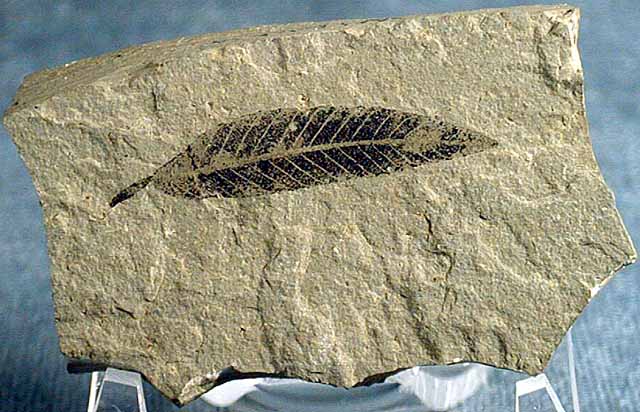In this image, we see a detailed depiction of a large, dark gray rock with a fossilized feather imprinted on it. The feather, which is black in color, features a single central vein with protrusions extending outward, resembling a V-shape. The fossilized feather is long and tapered, prominently displayed near the upper middle section of the rock. The rock itself is irregularly shaped with sharp points and grooves, and is situated on top of a blue piece of cloth adorned with white markings. The stone appears thick and has variations in its color, with darker and lighter patches adding to its texture. There is no text visible in the image, which focuses solely on the intricate details of the fossilized feather and the rugged, multi-toned rock.